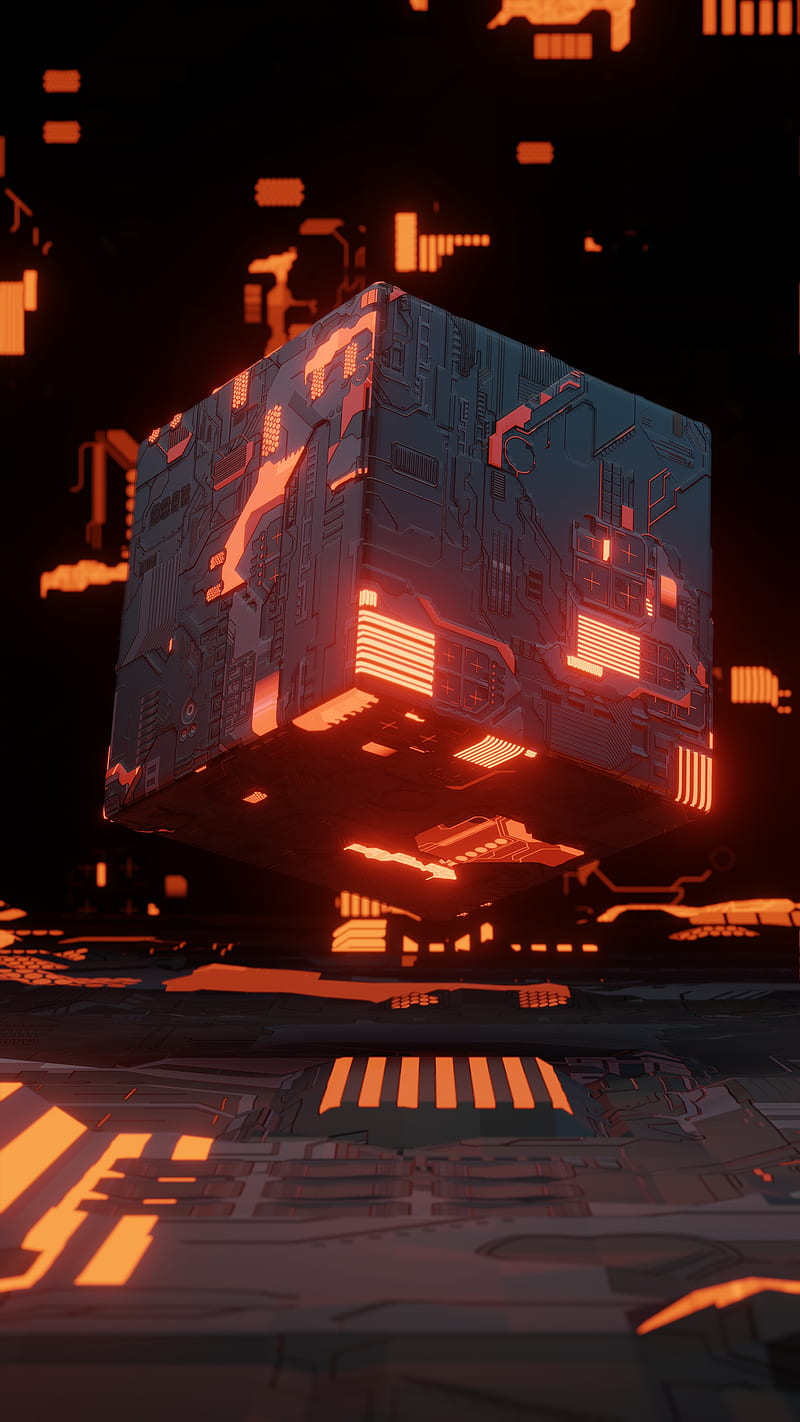This image showcases an abstract, futuristic, high-tech cube set within a cyberpunk-esque scene. The cube, rendered in dark gray and black tones, stands out against the background with vibrant orange LED highlights that form geometric patterns, reminiscent of circuit boards. Positioned at an angle, with its closest corner facing the viewer, the cube appears to hover above a ground similarly adorned with orange LED lines, evoking impressions of molten lava or molten steel. The background mirrors this high-tech aesthetic, creating a cohesive and immersive digital art piece. The scene's only light source, the orange LEDs, adds a striking contrast, further enhancing the cube's intricate, Star Wars-like design. Overall, the image blends themes of advanced technology and otherworldly elements, resulting in a captivating and detailed visual experience.